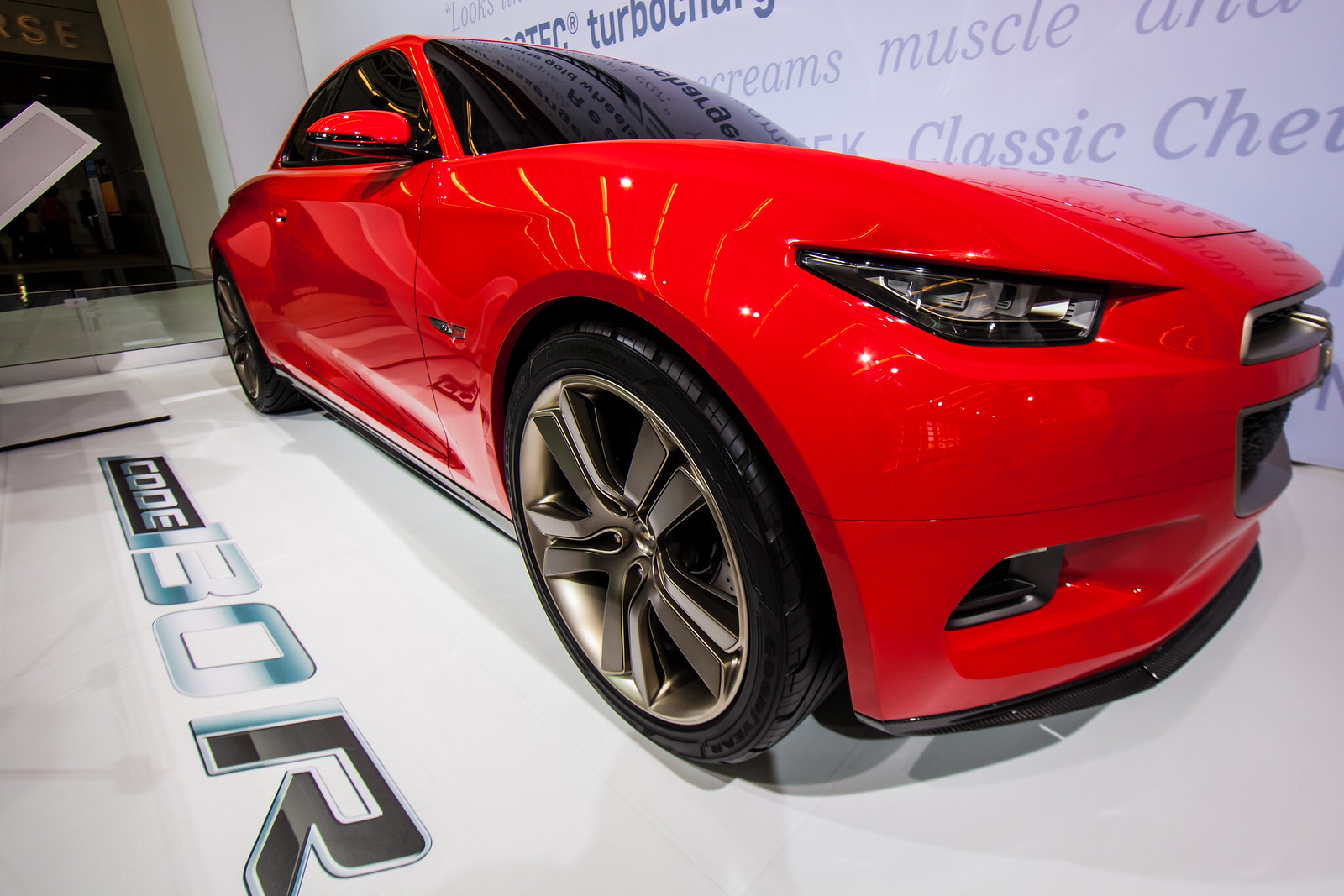The photograph features a striking bright red sports car, gleaming under the light. The car's surface is flawlessly smooth, showcasing its impeccable maintenance. The wheels are equally impressive, with shiny, pristine hubcaps that add to the overall aesthetic appeal. The brand new tires appear as though they have never been used, contributing to the car's impressive presentation. The dark, reflective windows mirror the surrounding environment, amplifying the car's polished look. Even for someone who isn't typically a car enthusiast, the vehicle's design is undeniably captivating. The sports car is a two-seater with a single pair of doors. On the ground parallel to the car, there is a text that reads "Code BOR."